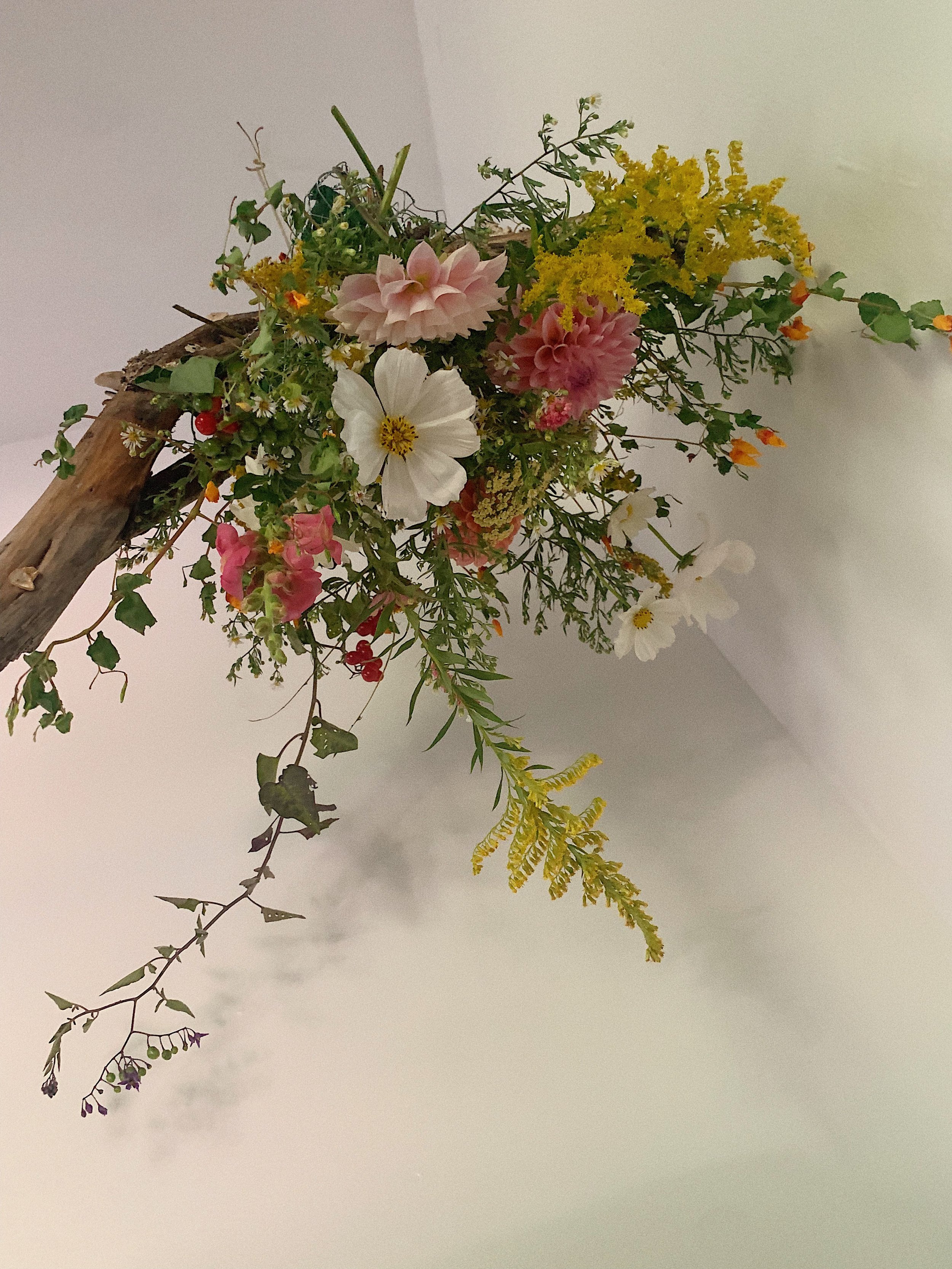The image depicts an indoor scene featuring an artful arrangement of various flowers and greenery against a pared-back, white backdrop. A smooth, pale brown wooden branch extends diagonally from the left side of the image, adorned with a lively mix of flowers and foliage. The vibrant display includes large flowers like a central white daisy-like bloom, a light pink flower positioned above it, and a deeper pink carnation to the right. Scattered throughout the composition are small white daisies, sprays of yellow blossoms, unopened orange buds, and flowers in shades of brownish-yellow. The greenery, consisting of both bright and dark green leaves, cascades gracefully from one end of the branch to the other, interspersed with delicate vines and what appear to be small red and orange berries. The arrangement sits upon a white and black table, enhancing the contrast against the white wall, giving the display a modern and minimalist aesthetic.